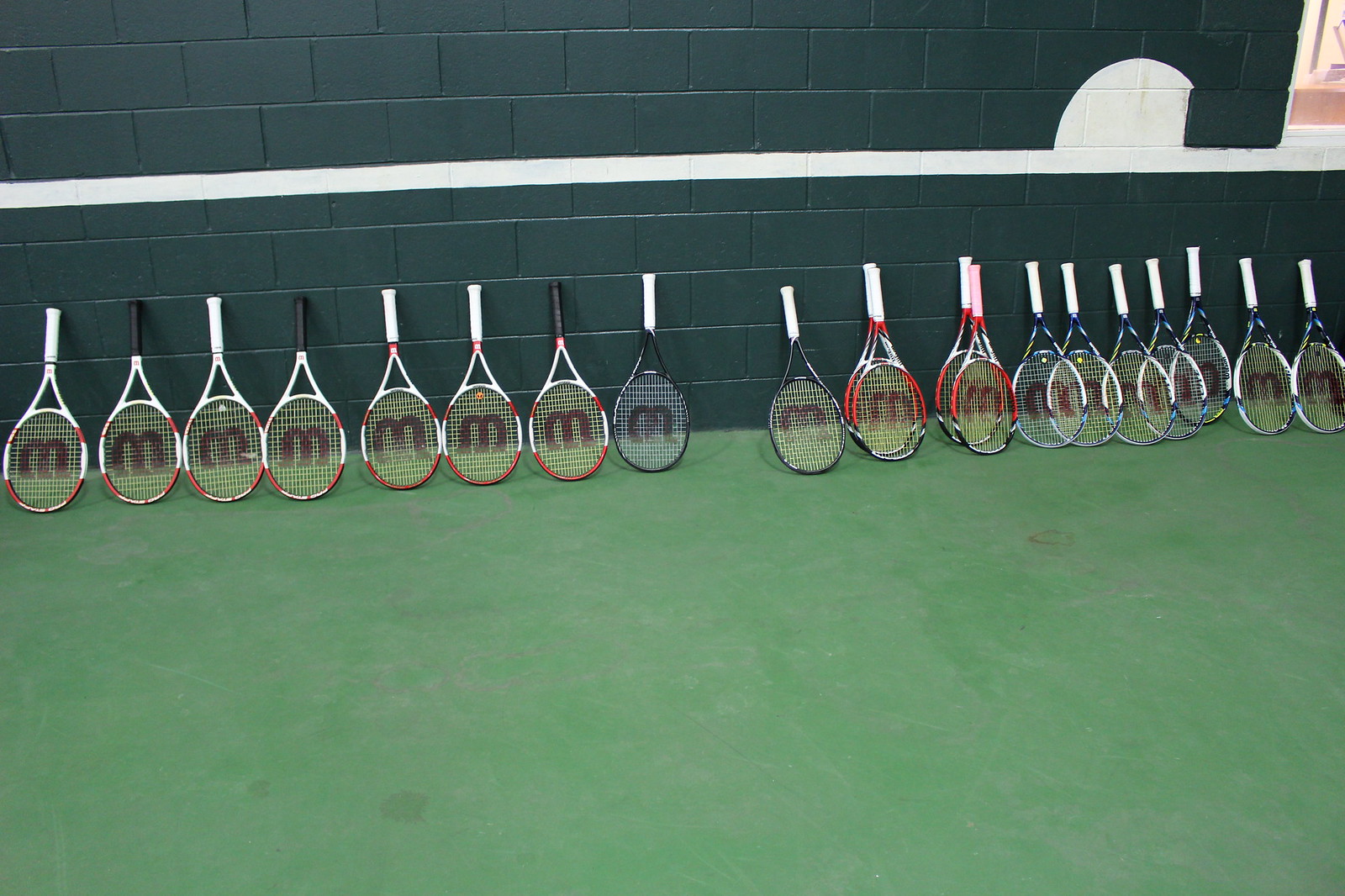This detailed photograph captures a striking arrangement of approximately 20 tennis rackets lined up against a deep forest green concrete block wall. These upside-down rackets, with their handles resting on the wall, are mainly wrapped in white tape, with a few featuring black tape. Each racket prominently displays a black "M" logo on the netting. The outer frames of the rackets show varying shades of dark red and light red. The green wall features a thick horizontal white stripe across its middle, and towards the right side, a white semicircle partially occupies two concrete blocks. The bottom of the image reveals a section of the tennis court, lighter green than the wall, indicating either green clay or a synthetic surface. The top right of the photograph hints at a background with hues of brown and tan, adding a subtle contrast to the scene.